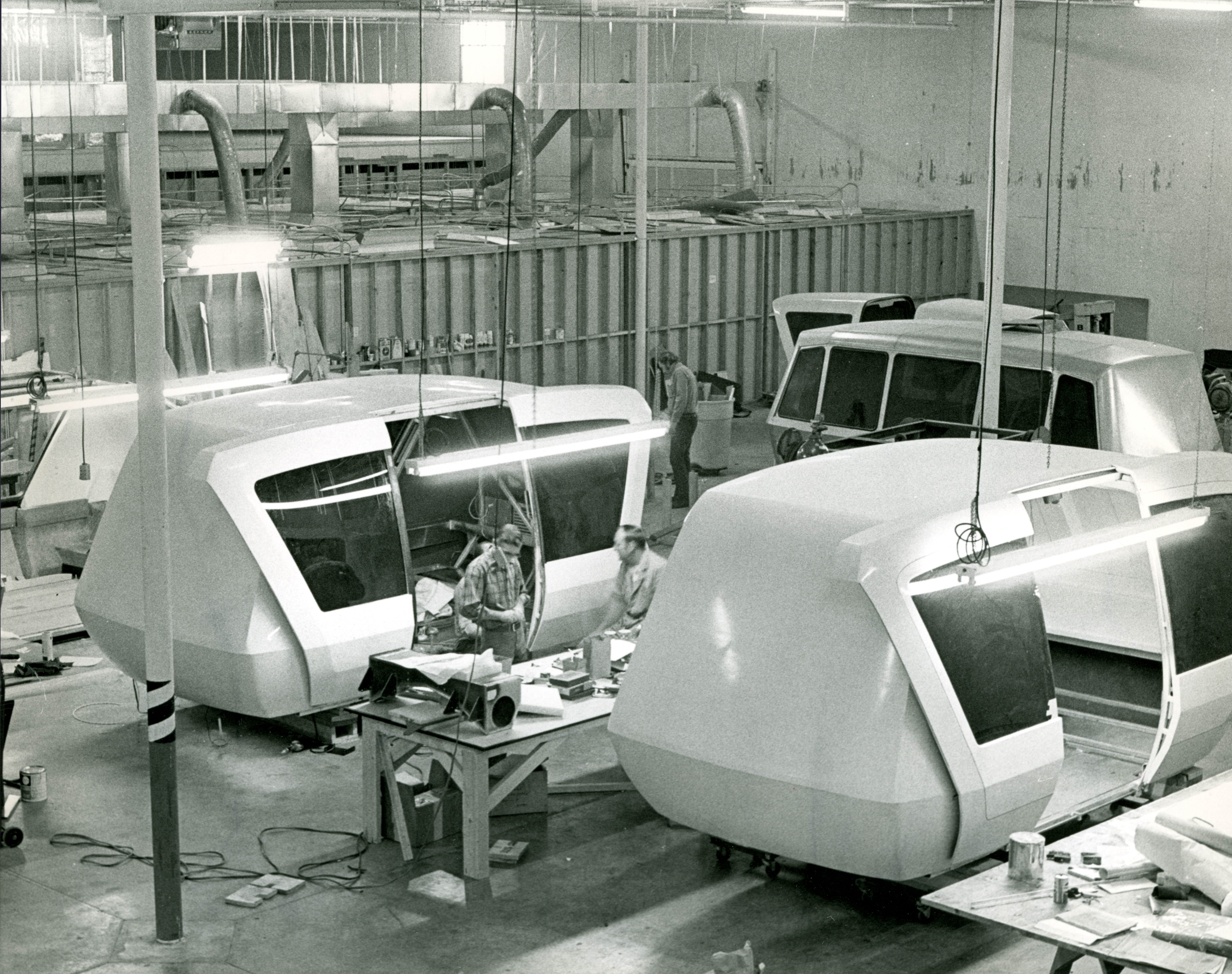The image is a large, square, black and white photograph taken inside a factory that captures an intricate scene filled with rich details. Central to the image are two men engaged in conversation, standing near a rectangular wooden table cluttered with various objects. The man on the left looks down, seemingly focused on the items on the table, while the man on the right speaks to him, gazing in his direction. 

Surrounding the men are several sizable, transportation-related structures that resemble oversized compartments of ski lifts or possibly components of a subway car or small rail vehicles. These structures have a rounded, somewhat oval shape, with their exterior appearing white or light gray, though the black and white nature of the photo makes precise colors ambiguous. Each structure features large, central windows with dark, see-through panels that split and open in the middle, sliding left and right.

The factory setting is further detailed with concrete flooring scattered with cords, and illuminated by fluorescent lights hanging from poles attached to the ceiling. Tall poles or pipes extend from floor to ceiling within the space, adding to the industrial atmosphere. The overall composition gives an impression of a busy work environment focused on assembling or manufacturing these unique transportation modules.